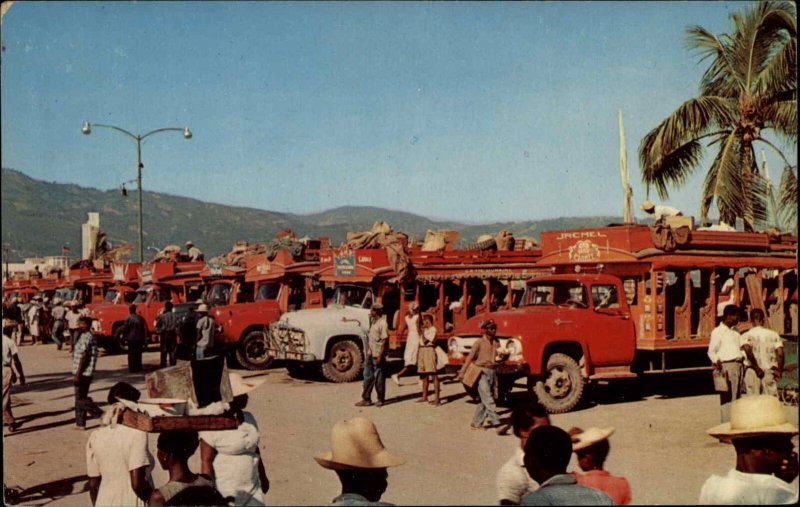This vibrant image captures a bustling outdoor scene in Jacmel, Haiti, likely from the 1960s or 70s. The sky is a clear blue, and lush green mountains rise in the background. A verdant palm tree stands prominently, casting a tropical feel. Lined up in the foreground are several trucks, predominantly red with a few white ones, loaded with supplies and people, possibly en route to work or the local market. 

A traffic pole with dual lights is visible amid the activity. The scene is alive with people dressed in various attire, including long sleeves, short sleeves, dresses, shorts, and skirts, accessorized with hats. Some individuals balance products on their heads, suggesting a vibrant marketplace atmosphere. A man, dressed in a white shirt, white hat, and black pants, stands atop an umbrella near the palm tree, adding a curious focal point to the tableau. Overall, the image exudes a sense of communal energy and daily life under the bright, welcoming sun.